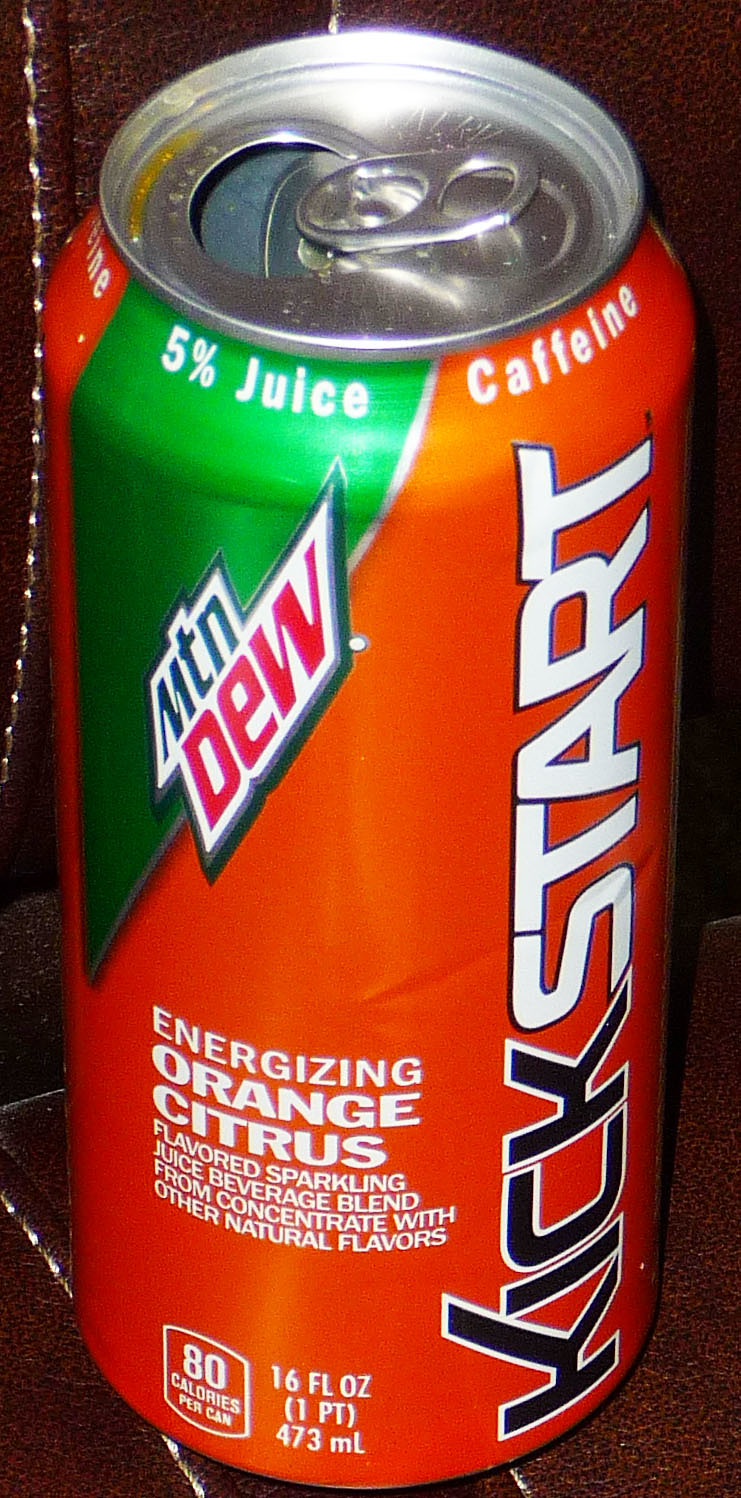This image features an aluminum can of Mountain Dew Kickstart. The tall, vertically oriented photograph has been trimmed to focus exclusively on the can, which is placed on a brown leather couch with visible white stitching. The top of the can is popped open, revealing a pull ring on the right-hand side and an opening to the left. The can itself is primarily orange with a distinctive green stripe descending from the rim down to the middle left side. 

Near the top rim on the green stripe, the text "5% Juice" is prominently displayed, while "Caffeine" is marked on the orange part of the can. The iconic Mountain Dew logo is placed in such a way that it partially overlaps the green stripe. Running vertically down the can, the word "Kickstart" is boldly printed, with "Kick" in black and "start" in white. Adjacent to this, the flavor description reads: "Energizing Orange Citrus Flavored Sparkling Juice Beverage Blend From Concentrate With Other Natural Flavors."

The background, with its textured leather and stitching, provides contrast to the vibrant colors of the can, making it the focal point of the image.